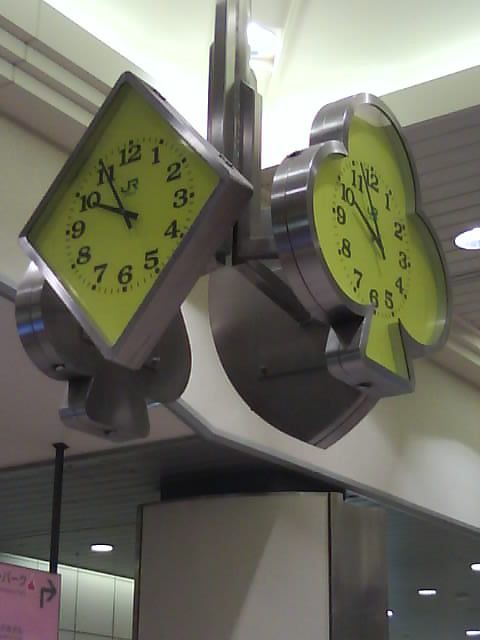The image depicts a bustling transportation terminal, possibly a bus or train station, characterized by a sleek, industrial design. The ceiling is recessed and features abundant recessed lighting, giving the space a modern ambiance. Prominent structural elements are predominantly metal, contributing to the terminal's sturdy and contemporary aesthetic. Suspended from a strong silver support high up in the open ceiling, which appears to have a skylight allowing sunlight to permeate the space, are four clocks. Each clock presents a different face, reminiscent of playing card images: the back of the heart suit, the club suit facing forward, the diamond suit facing forward, and the back of the spade suit. The clocks have green backgrounds with black numbers, adding a touch of color to the metallic environment. Below, the terminal floor is lined with pristine white tiles, and the area is accented with a variety of metal elements. A notable feature is a pink sign with an arrow, serving as a directional guide for travelers.